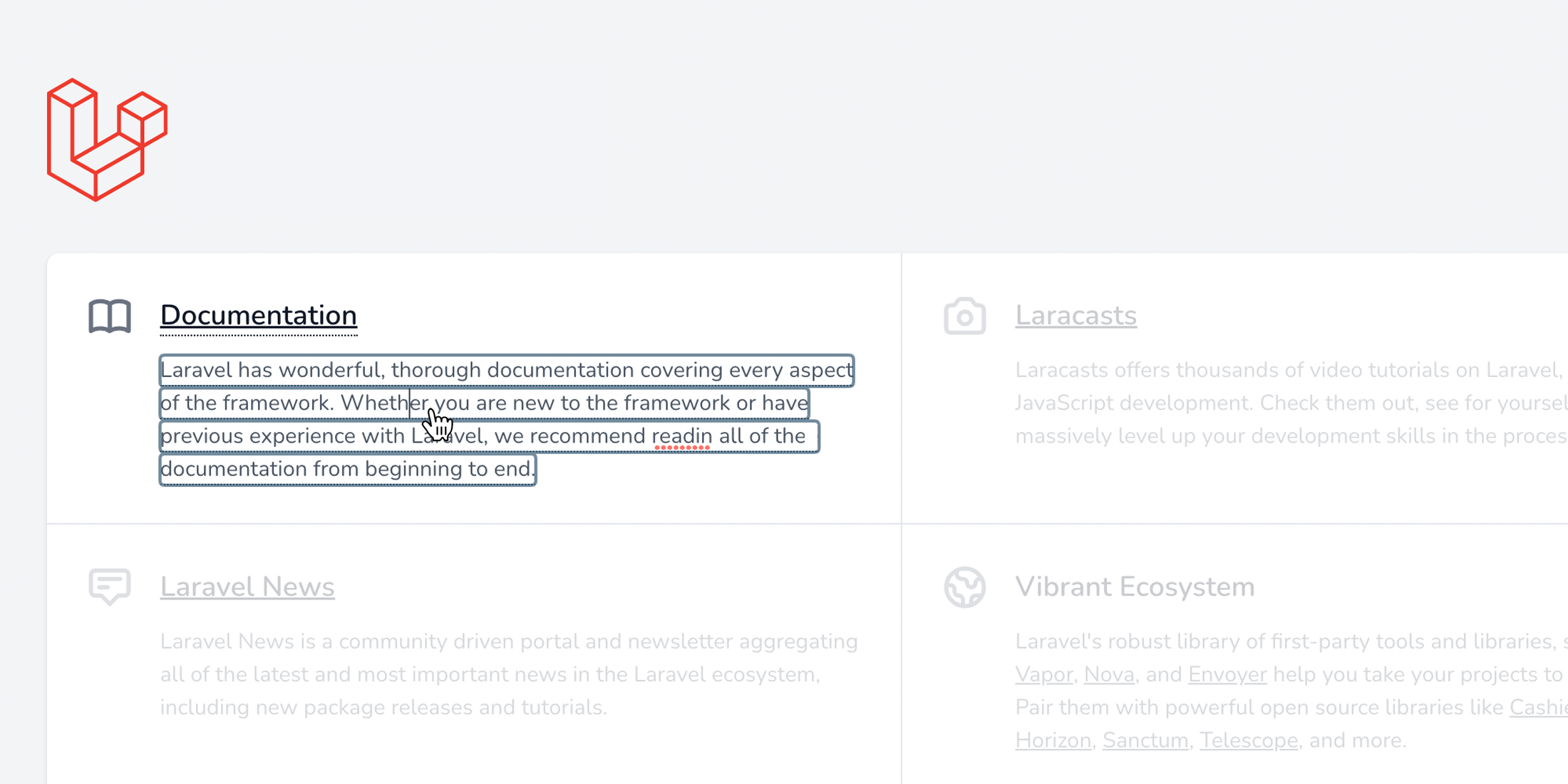The image captures a screenshot from a document system related to Laravel. The top left corner features a logo comprised of a set of blocks resembling Legos, outlined in red. This logo forms an L-shape with an additional block attached precariously to one edge, giving the impression it might fall off.

Below the logo, there's a highlighted section accompanied by a book icon. The highlighted text reads: "Documentation. Laravel has a wonderful, thorough documentation covering every aspect of the framework. Whether you are new to the framework or have previous experience with Laravel, we recommend reading all of the documentation from beginning to end."

Following this highlighted section, the text turns gray, with the next section titled "Laravel News" stating: "Laravel News is a community-driven portal and newsletter aggregating all of the latest, most important news in the Laravel ecosystem, including new package releases and tutorials."

Additional grayed-out sections are titled "LarCasts" and "Vibrant Ecosystem." The "Vibrant Ecosystem" section elaborates: "Laravel's robust library of first-party tools and libraries. Vapor, Nova, and Envoyer help to take your projects to pair them with powerful open source libraries like Cache, Horizon, Sanctum, Telescope, and more."